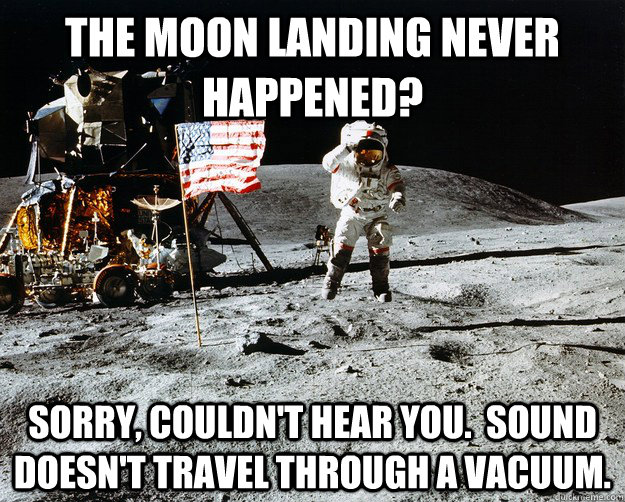The image depicts a heavily muscular, middle-aged, bald man lying shirtless on a bed, displaying a salt-and-pepper beard and mustache, along with a prominent tattoo on his right shoulder. He wears a black and grey belt around his waist with a strap on his right thigh, and is not wearing any pants. His strongly built arms press down on the bed, centered around a black cylindrical object with a white ribbon sticking out from his midsection. The bedspread features a camouflaged pattern in red, grey, white, and black, with the word "HIGH" in large, white, capital letters at the bottom of the image. Behind him are two black pillows with white ribbons, complementing a dark blue wall in the background. The bedposts, made of dark wood, ascend beyond the top edge of the photograph, framing the scene.